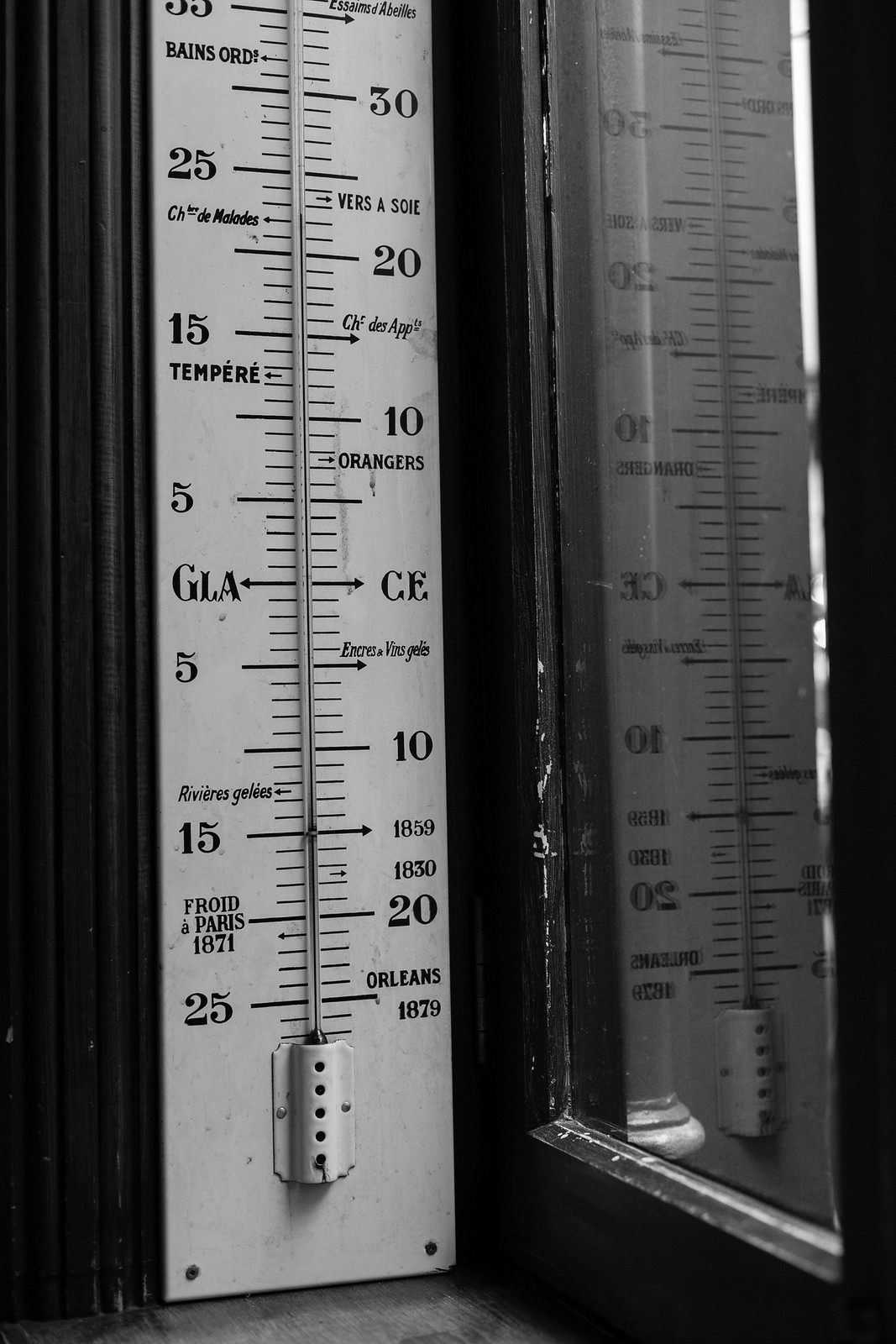This image showcases a vintage thermometer with an intricate white face, possibly made of metal or wood. The thermometer features black lines and numbering to mark different temperatures. A slender mercury tube ascends through the center of the face. On the left side, the numbers are organized in descending order: 25, 15, and 5, with the abbreviation "GLA" noted at the center. The right side numbers follow a similar pattern: 30, 20, and 10, with "CE" opposite "GLA" in the middle. At the bottom of the thermometer, the text reads "Orleans 1879."

Additional lettering includes "Freud to Paris" positioned between the 25 and 15 on the left, and "Orangers" just under the upper 10 on the right. There are other inscriptions on both sides, though they are not fully legible. The thermometer is displayed against a wall surface, possibly leaning near a window sill. The nearby window pane, framed in black, provides a faint reflection of the thermometer's setup. This amalgamation of details points to a carefully crafted and historic piece.